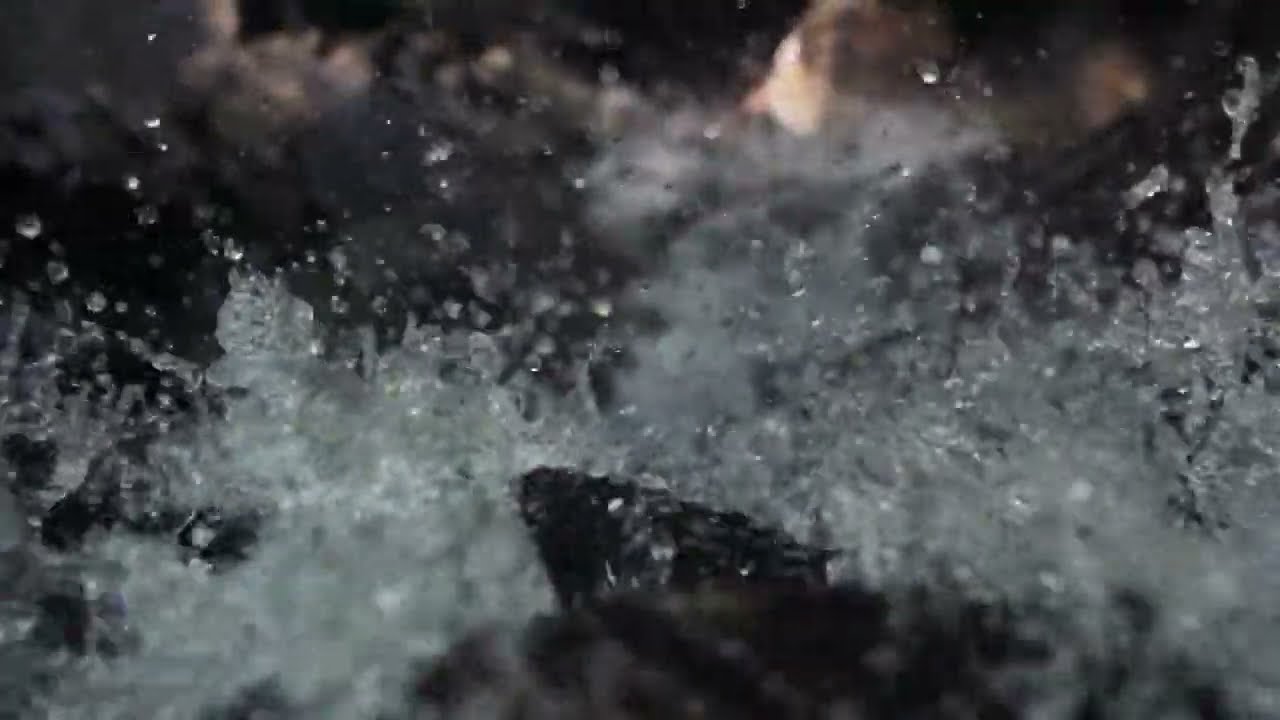The landscape-oriented image depicts a dynamic, freeze-frame moment of water forcefully splashing over dark, gray rocks. The water appears as a cascade of individually captured droplets, creating a sense of motion frozen in time. The rocks in the foreground form a rough triangle, with water shooting up and over them, vividly contrasted in shades of white and gray. The background rocks appear blurred and varied in color—dark gray and light—adding depth to the scene. Despite the uncertainty of whether the image is real or computer-generated, the detailed elements like the fine water droplets and the realistic portrayal of the rocky formations give it a strikingly realistic appearance. Additionally, there seems to be an indistinct hole or an opening in the background rocks, possibly indicating daylight filtering through. The detailed focus on the foreground adds to the sense of action and realism, embodying a snapshot of vigorous natural motion.